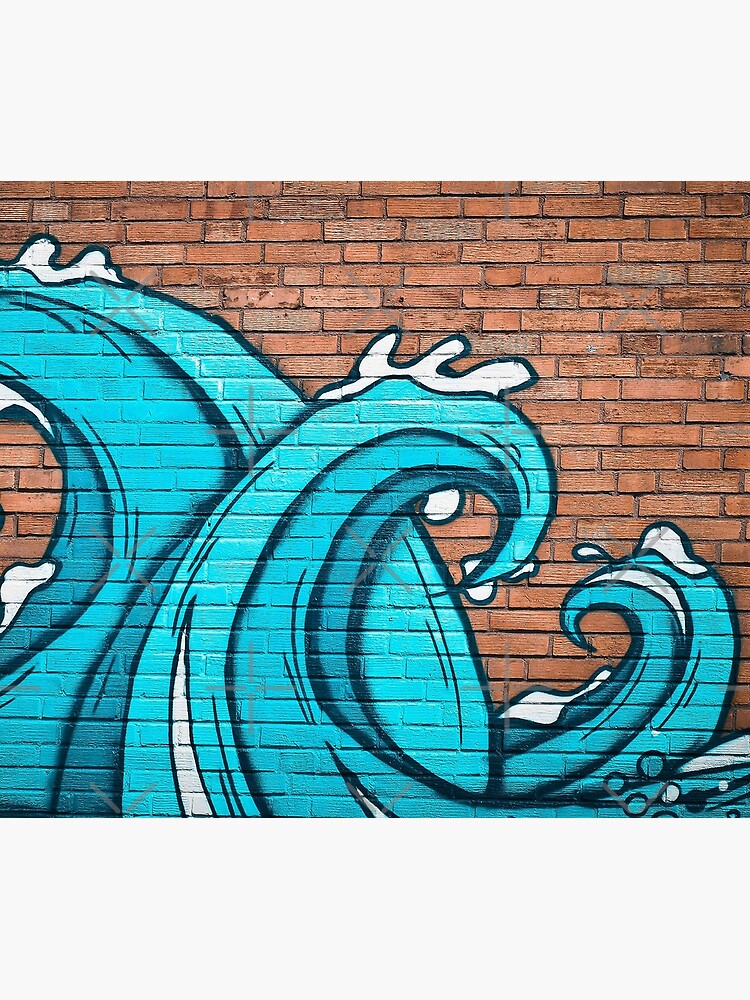This rectangular image, measuring approximately six inches in height and four inches in width, features a light gray border about an inch thick around all sides. At the center of the image, there is a photograph taken outdoors during the daytime, capturing a reddish-brown brick wall with darker red grout. The focal point of the photograph is a mural in progress, depicting a dynamic scene of curling ocean waves.

The mural reveals three prominent waves, each distinct in size and direction. The first wave starts from the bottom left corner, extending to the center right, before curving upwards and back to the left, adorned with black lines indicating motion and white foam caps. The second wave emerges from the lower right corner, trailing low along the bottom before rising and curling towards the top and center right, showing a dramatic arc and white-tipped crest. The smallest of the waves is situated in the lower right corner.

Additional details include gray X's scattered across the entire image, serving as a watermark. The waves are painted in varying shades of blue, from light to dark, with intricate white foam details, evoking the motion and energy of the ocean against the backdrop of the brick wall. The combination of these elements creates a vivid and animated scene, capturing both the artistry and the natural beauty of ocean waves.